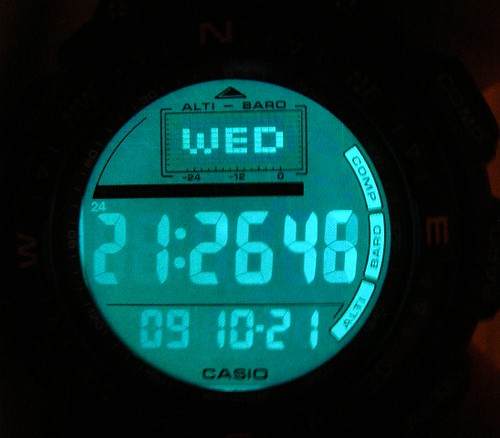This is a close-up, portrait-style photograph taken in the dark, focusing on an illuminated digital Casio watch. The round face of the watch, which occupies about 80% of the square image, glows in a pale blue hue, with the numbers and other details highlighted in a brighter light blue. The time displayed is 21:26:48, with the date 09-10-21 shown directly beneath it. At the top of the face, above the time, is the abbreviation "WED" for Wednesday, alongside the word "ALTI-BARO." The lower part of the face prominently features the brand name "Casio" in black letters. The watch's face is flanked by three illuminated sections marked "COMP," "BARO," and "ALTI" against a white background. The entire setup is set against a completely black background, emphasizing the glowing details of the watch.